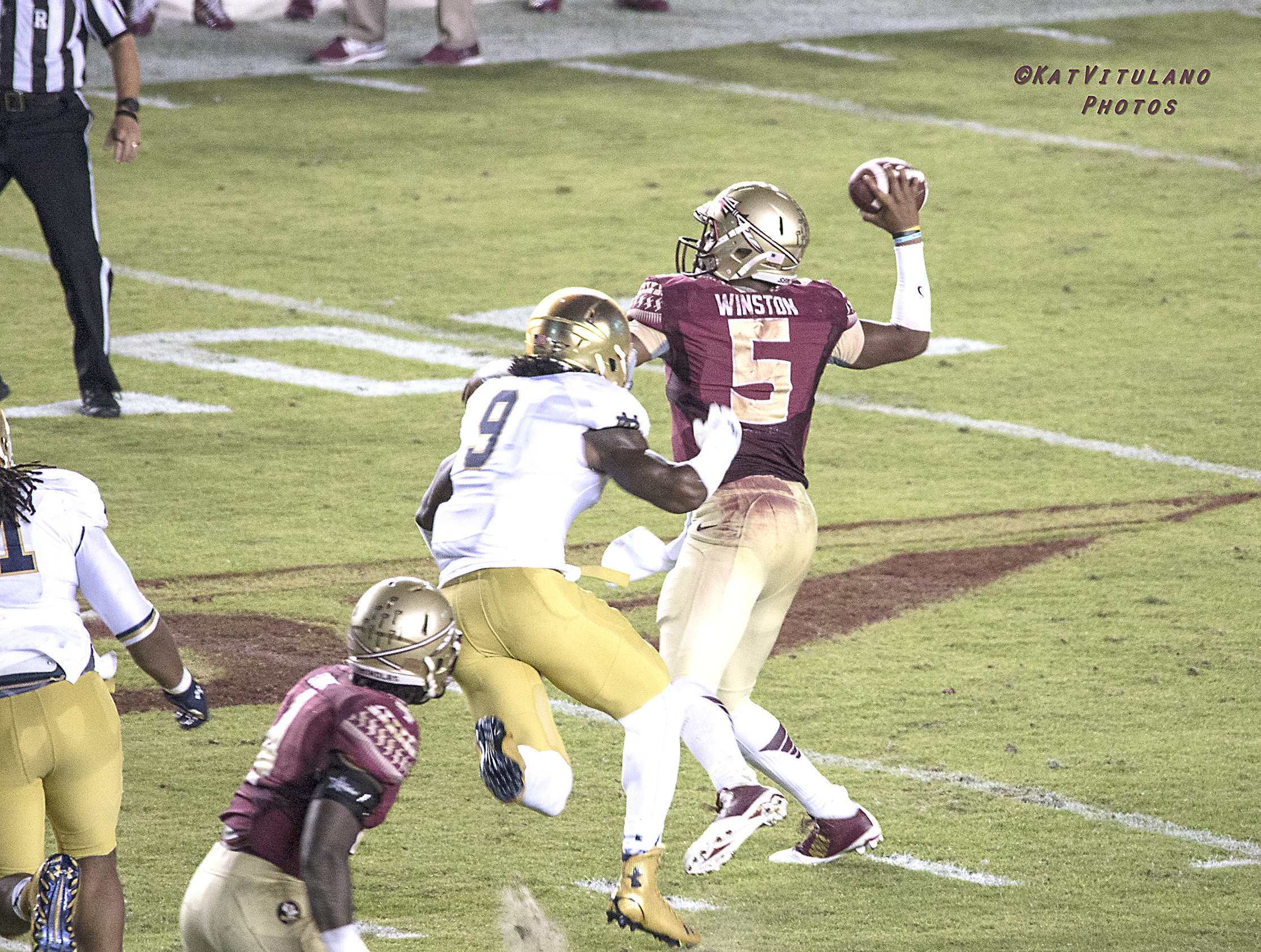In this captivating photograph of an NCAA college football game, the atmosphere is electric as Florida State University's quarterback, Jameis Winston, prepares to throw the football. Dressed in a red jersey emblazoned with 'Winston 5' in white letters, paired with gold pants and a matching gold helmet, Winston is visually striking against the lush green field marked with bold white lines. As he initiates his throwing motion, a player from the opposing team, potentially Central Florida, rushes toward him. This defender wears a white jersey with the number 9, gold pants, white socks, gold sneakers, and a gold helmet. Both players are black, emphasizing the diversity on the field.

The intensity of the moment is further highlighted by another Florida State teammate in the background, similarly clad in red and gold, whose number remains obscured as his back is turned to the camera. In the bottom left-hand corner, another opposing team player in a white and gold outfit adds to the scene's dynamic nature. The top left reveals a portion of a referee, donned in a classic black and white striped shirt with black slacks and a white stripe, overseeing the play. The background also features the cutoff feet of players, identifiable by their red sneakers, hinting at the broader team's presence.

The setting appears to be a nighttime game, illuminated by powerful stadium lights. Completing the image, the top right-hand corner bears the watermark 'copyright Cat Vitulano Photos,' asserting the photographer's credit. This detailed scene encapsulates the high stakes and fervor of college football, capturing a crucial moment in Jameis Winston's career at Florida State University.